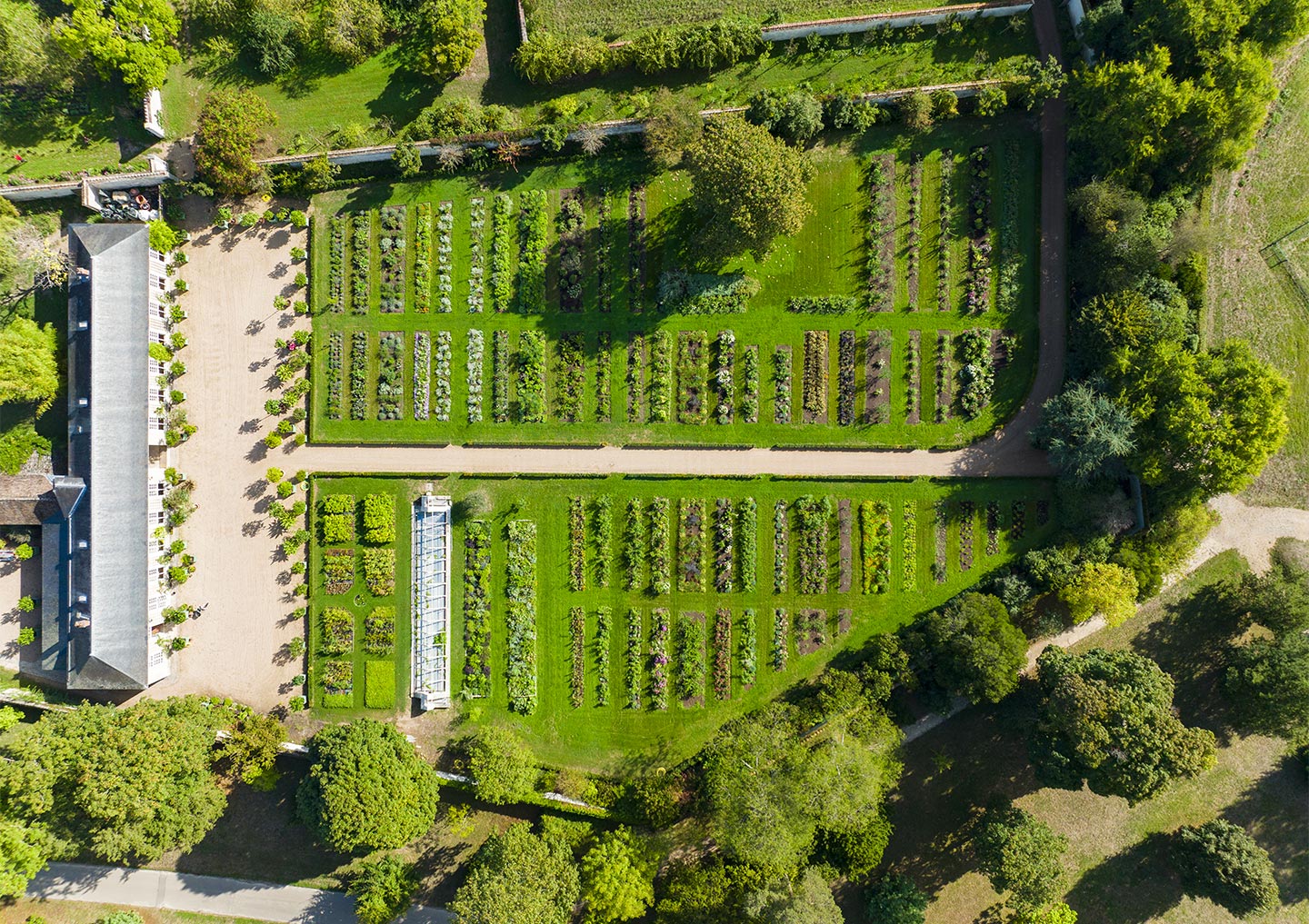This aerial photograph captures a detailed view of a large outdoor field, predominantly featuring expansive green grass. Positioned on the left side of the image stands a notable long white building with a gray roof, fronted by a substantial concrete plaza. This building, seen toward the top left of the view, is bordered by a distinct boundary wall. Within the field, there are neatly sectioned rectangular planted beds, suggesting a well-organized garden setup. These beds are separated by a single row walkway that traverses the area, moving from one end to the other before curving upward towards the end. Enhancing the scene, the field is fringed by an array of trees, which enclose and separate it from the adjacent green fields, contributing to the structured and verdant landscape. The variety of plants and the organization within the garden adds vibrant colors to the predominantly green scenery.